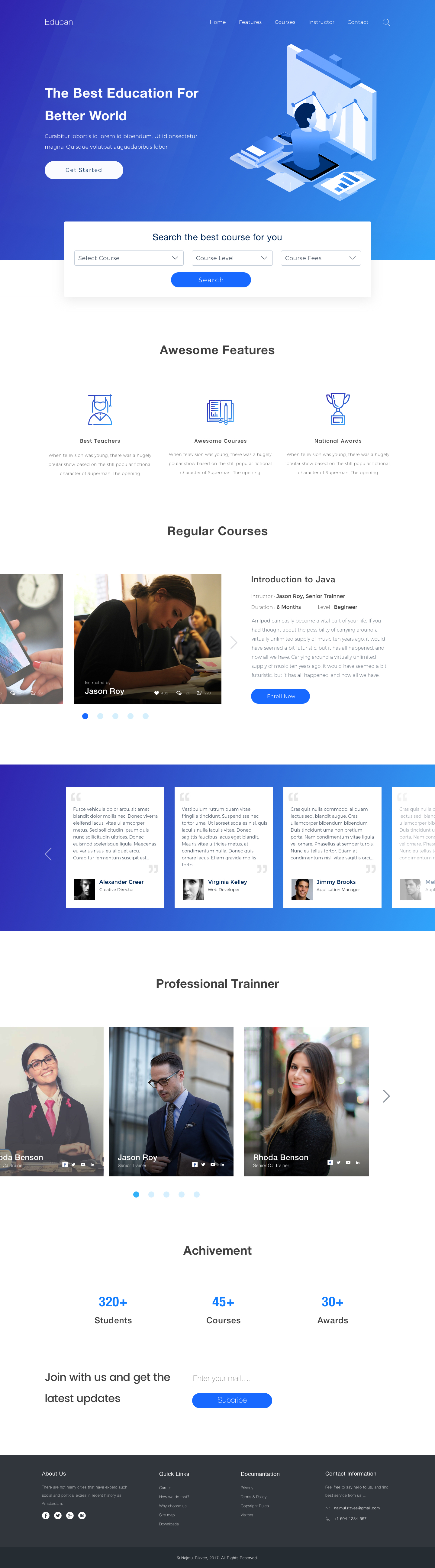Here is the detailed caption:

"This is a screenshot of a slightly low-quality and blurry website. At the very top, a blue rectangle with white font proclaims 'The Best Education for a Better World.' Below this, there is a line of smaller white text that is not legible. Beneath that, a white oval contains blue text, also unreadable.

To the right of this text, there is an illustration of a person emerging from a flat-screen monitor. The depiction shows only their upper torso, and they are focused on examining a bar graph displayed on a whiteboard in front of them.

Below this graphic, a white search field is visible. Directly below the field, 'Awesome Features' is written in black font. Underneath this heading, there are three small icons. The icon on the far right resembles a trophy, while the other two icons are not identifiable.

Further down, the text 'Regular Courses' appears in black font. Below this, there is an image of a woman intensely writing in a notebook at a desk. She appears focused and determined.

At the bottom of the screenshot, there's a white bar containing white text that looks like user testimonials."